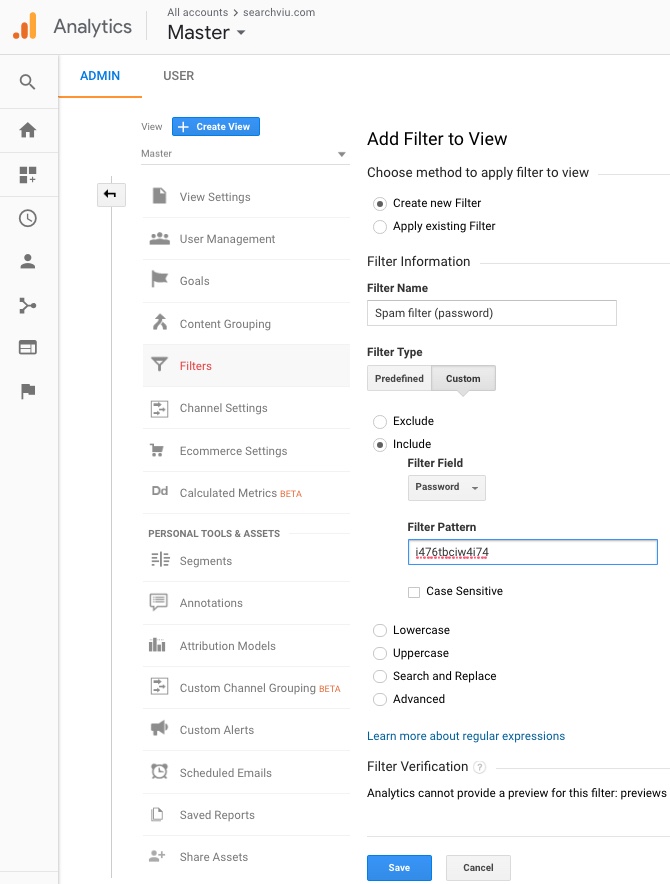This image showcases the internal settings page of a programming or analytics application, displayed in portrait orientation. The design is primarily against a white background with a grey vertical border on the left side and a horizontal border at the top.

In the top left corner, there is a chart-like graphic labeled "Analytics," composed of three orange bars in ascending order of size and brightness. To the right of the chart, the text reads "All Accounts Master."

Running down the vertical gray column on the left side are various icons, including a magnifying glass, home, clock, and others, indicating different navigational options.

Within the main white box of the interface, the word "Admin" is highlighted in blue with an orange underline, while the word "User" remains unselected in gray.

Below this, the interface displays the word "View," followed by a blue button labeled "Create View" with a white plus sign. Various drop-down menus are available underneath this button, offering options such as "View Settings," "User Management," "Goal," "Content Grouping," and "Filters."

To the right, another section allows for adding filters to the view. Text prompts include "Add Filter to View," "Choose Method to Apply Filters to View," "Create New Filter," "Apply Existing Filter," "Filter Information," and "Filter Name."

At the bottom of the page, there are two buttons: a blue "Save" button and a white "Cancel" button, allowing users to either save their settings or cancel the operation.